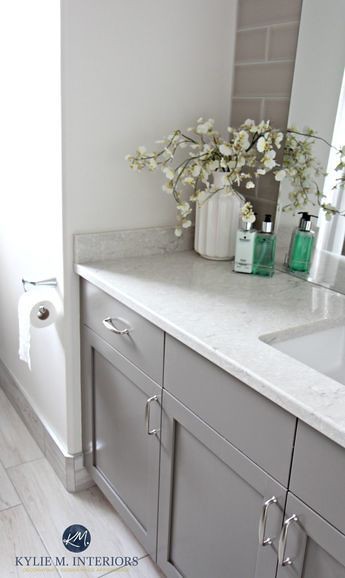A meticulously designed bathroom showcases a harmonious blend of white and gray tones, accented with subtle pops of green flora for a touch of nature. The pristine white walls and elegant gray vanity—with its matching gray shelves and drawer facades—create a sophisticated, monochromatic ambiance. Adding to this serene palette, the vanity features sleek stainless steel handles and a marbled countertop, elegantly combining shades of white and gray. 

On the vanity counter, a stylish green soap pump bottle adds a splash of color, complemented by a white ceramic pot containing a delicate plant with white petals and green leaves. The sink is seamlessly integrated into the marbled surface, enhancing the bathroom’s streamlined look.

The backsplash behind the vanity is composed of gray tiles, providing a textured contrast to the smooth surfaces elsewhere. The gray tile floor, adorned with subtle whitish streaks, ties the entire color scheme together. To the left, a roll of toilet paper is mounted on a wall holder, hanging away from the wall for easy access.

In the lower left corner of the image, a black circular logo for Kylie M Interiors is visible, featuring the initials "KM" in a stylized white script. This thoughtfully designed space reflects both functionality and minimalistic elegance.